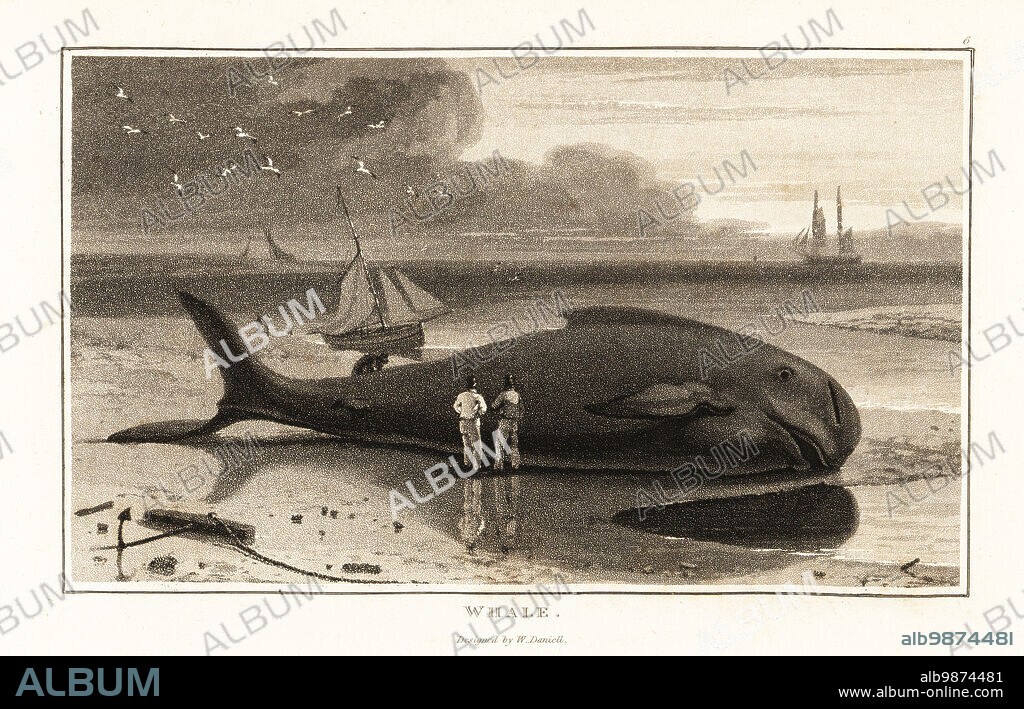This black and white illustration, possibly a combination of charcoal and ink, depicts a dramatic scene of a beached whale lying horizontally on a shore, framed by a thin, slightly brownish border indicative of its age. The whale, of a dark gray to almost black color, is the central focal point, lying with its massive body casting a shadow onto the adjacent water. Near its side, two men, dwarfed by the whale's size, are seen examining it, potentially conversing. Another smaller figure appears on the whale's opposite side, seemingly engaged in some activity.

The background reveals a seascape with darkening waters, seagulls, and several ships, suggesting a whaling operation. One ship, equipped with numerous sails, sits closer to the shore, while larger ships loom in the distance. The sky above, predominantly clear, has clouds adding a somber tone.

Notable on the beach is an anchor nestled into the sand, its chain running along the shore and potentially linked to the whale. Scattered rocks interrupt the mainly sandy beach, enhancing the rugged scene. Small details like the possible expression on the whale’s face add emotional depth, suggesting it might still be alive.

Watermarks and inscriptions provide context: it’s part of an album, with text such as "Whale, designed by W. Daniel" and codes like ALB9874481, alongside the website www.albumonline.com. Overall, the image captures a poignant moment in maritime history, blending human and natural elements in a powerful composition.